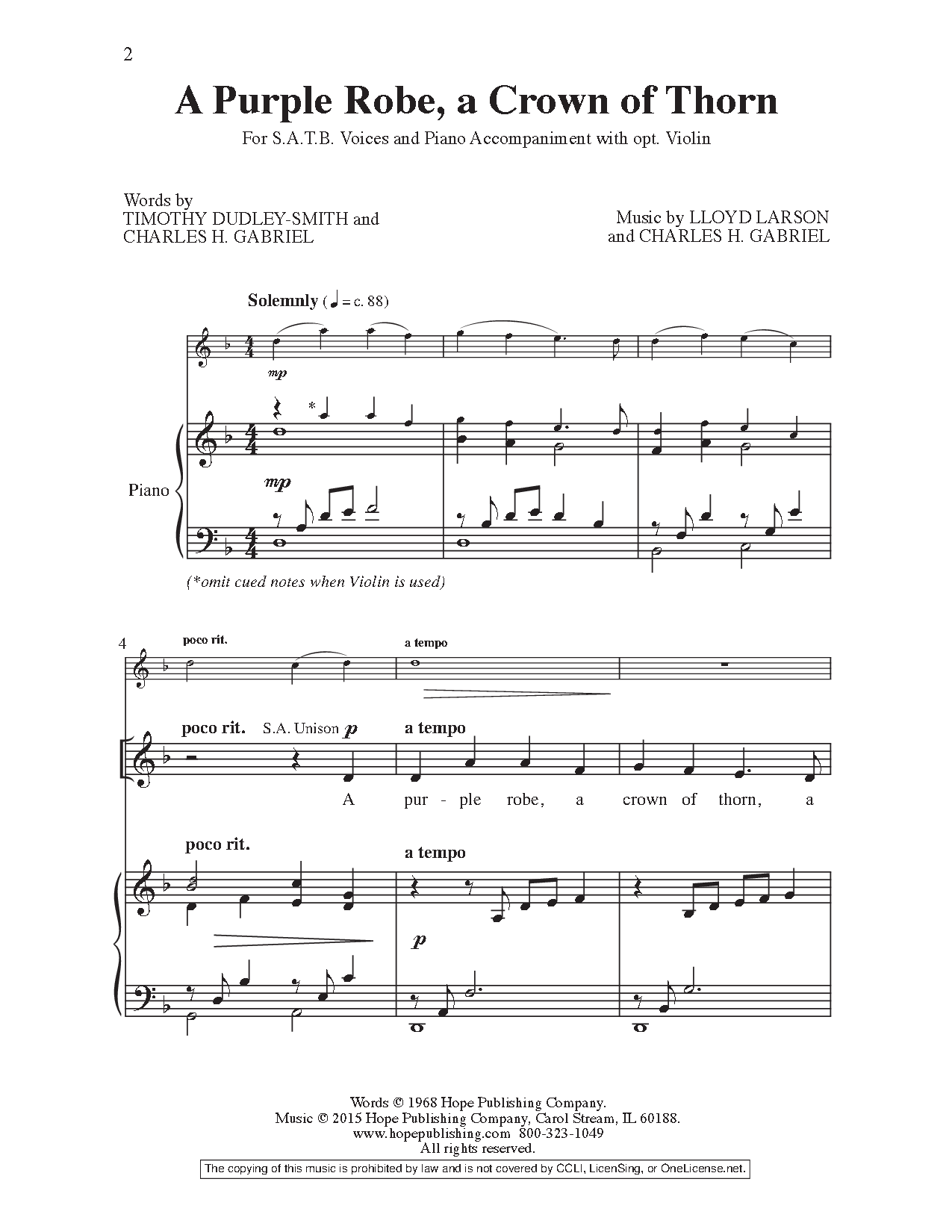The image is a digital screenshot of a page from a music sheet, presented on a white background. The page number "2" is located in the upper left-hand corner. The title of the piece, "A Purple Robe, A Crown of Thorns," is prominently displayed in a bold, serif font, most likely Times New Roman. Below the title, in a smaller font, the arrangement specifies "for SATB Voices and Piano Accompaniment with Optional Violin." SATB stands for soprano, alto, tenor, and bass.

On the left side of the page, it credits the words to Timothy Dudley-Smith and Charles H. Gabriel, while on the right side, it attributes the music to Lloyd Larson and Charles H. Gabriel. The body of the page contains musical bars and notes, with the top smaller set likely for the piano and a larger set at the bottom. At the very bottom of the page, it states, "Words copyright 1968 Hope Publishing Company. Music 2015 Hope Publishing Company, Carol Stream, Illinois," followed by the website "www.hopepublishing.com" and a phone number.